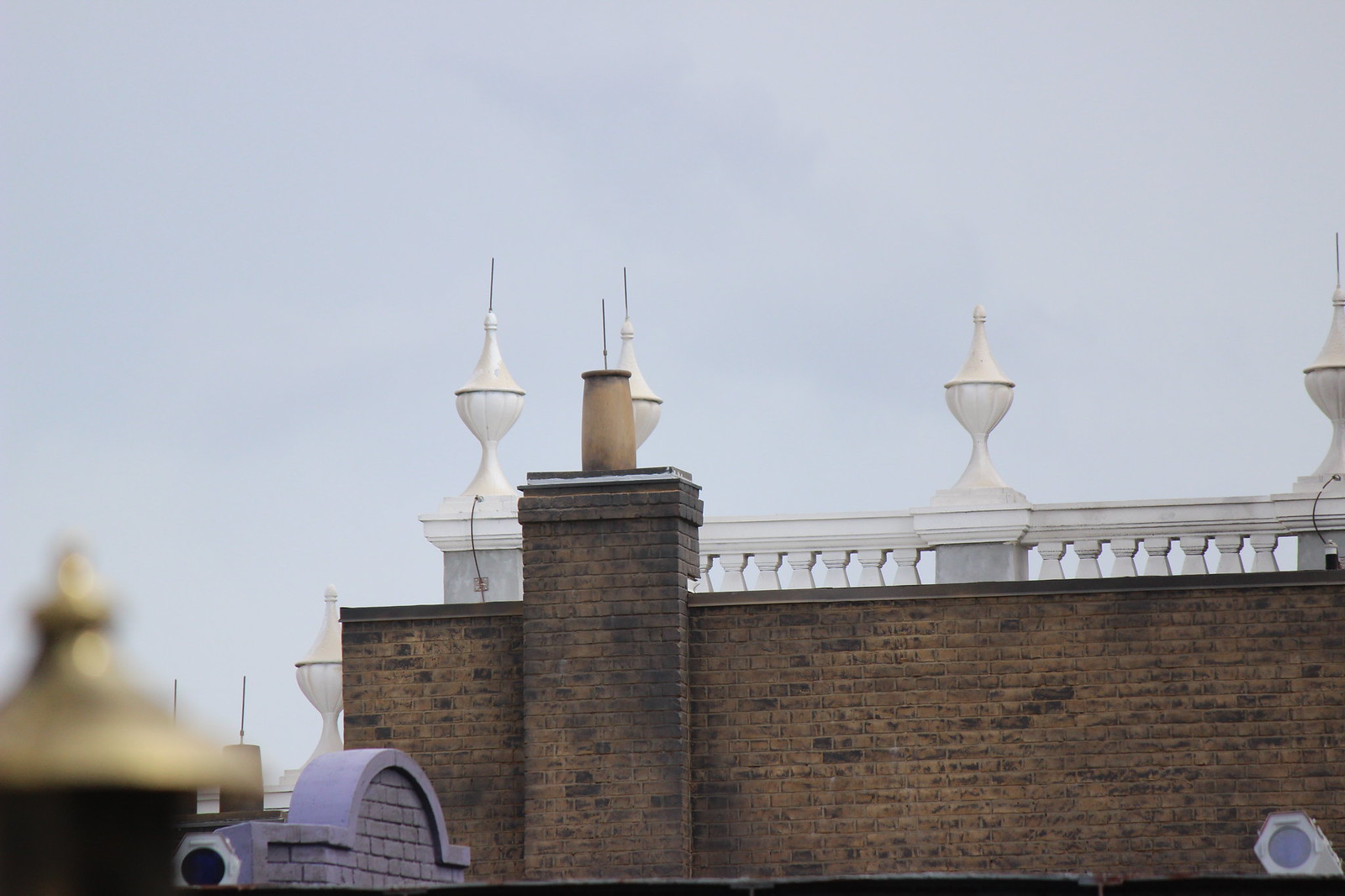The photograph captures the upper part of a weathered, red-brick building with dark, almost black, distressed bricks. The architectural style suggests an older European structure, possibly located in Ireland or England. A prominent white stone fence with thick, tapered spindles and ornate details runs horizontally across the building's roofline. Interspersed along the fence are statues resembling lidded chalices or urns with pointed tops. In the left foreground, there is a blurred, gold, bell-shaped element, its exact nature hard to discern, adding a touch of mystique. The background shows another building with gray bricks and an archway adorned with intricate molding, all set against a somber gray sky. The combined elements of the detailed brickwork, aged patina, and elaborate rooftop decorations create a richly textured and historical atmosphere.